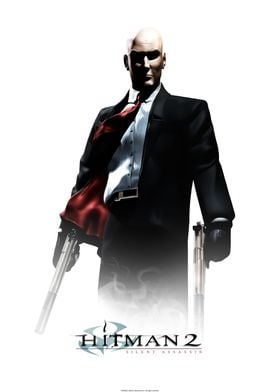In the image, set against a white background, is an animated portrayal of a bald man dressed in a dark suit, with a white button-down shirt underneath. The ensemble is accented by a red tie that appears to be waving slightly to the left. The man, who appears fair-skinned, has a sinister, shadowed facial expression, emphasizing a more menacing look. He is wearing black gloves and holding two shiny, metallic handguns with silencers pointed down at his hips. Notably, there is a maroon detail inside his jacket visible on his right side. Beneath him in the center of the image, the title "Hitman 2" is displayed in black text, underlined in grey, with some small writing beneath it. This image is identified as the cover art for the video game "Hitman 2," a game centered around an assassin.